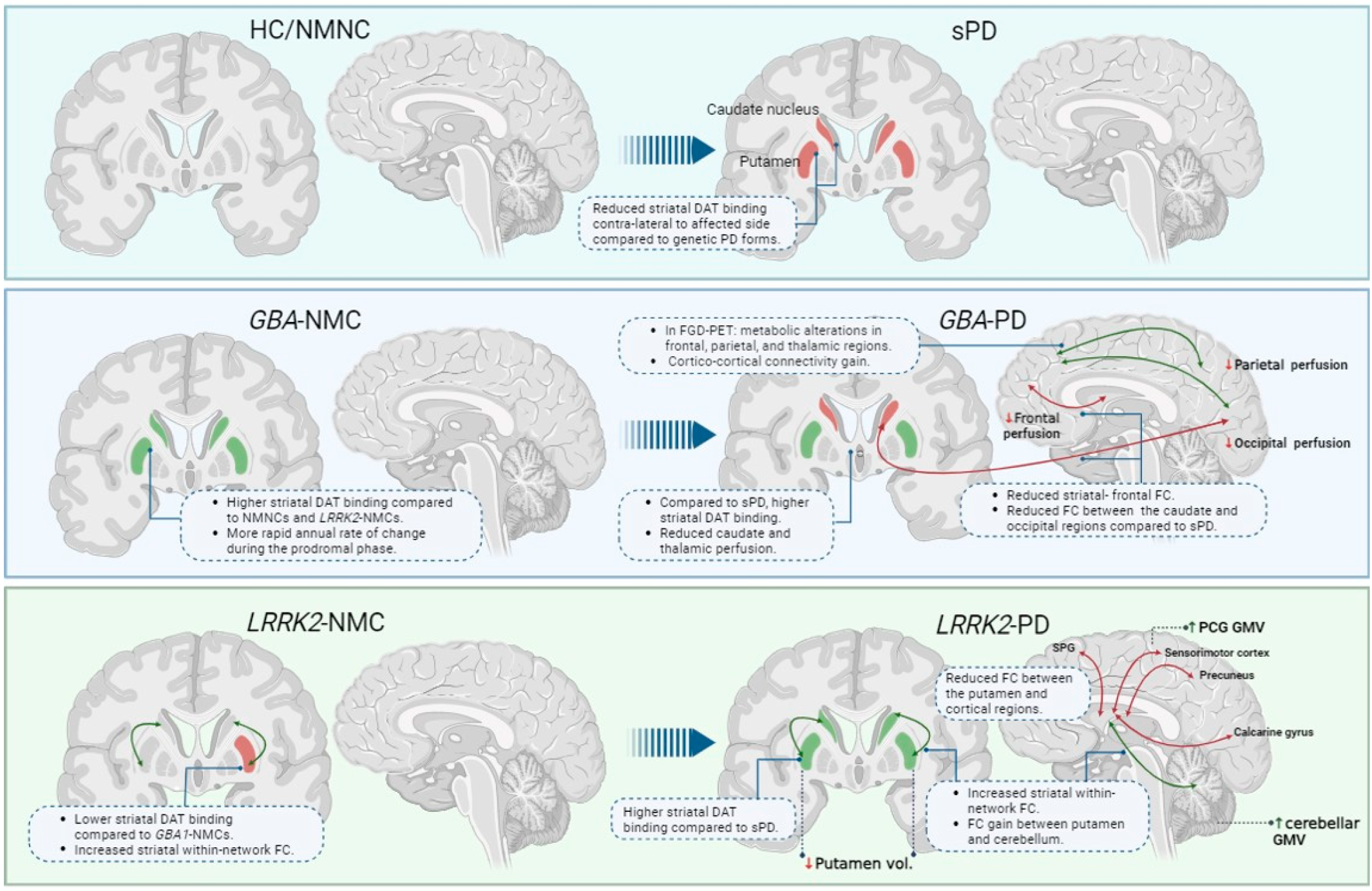This digital illustration comprises twelve detailed cross-sectional images of the brain, arranged in three horizontal panels on a very light blue background with darker blue borders. The top panel, labeled “HC/NMNC,” displays cross-sections of a normal brain, highlighted with gray illustrations and specific notations like "SPD" and "caudate nucleus putamen." This section also notes "reduced striatal DAT binding contralateral to the affected side compared to genetic PD forms." Green and blue arrows direct attention across the images, with a small, blurry explanatory box providing additional context.

The middle panel, tagged “GBA-NMC,” transitions into “GBA-PD” with illustrations showing areas of the brain in various colors, primarily green and red, indicating different levels of striatal DAT binding. The presence of arrows facilitates a comparison between the two states. The panel includes unclear small boxes of text that appear to offer detailed explanations, culminating in mentions of "partial perfusion."

The bottom panel, labeled “LRRK2-NMC” and “LRRK2-PD,” shows brain cross-sections with highlighted regions marked by green and red areas, indicating possible differences in brain activity or pathology. Arrows and additional small text boxes in this panel are also challenging to read but are intended to explain the specific differences and locations highlighted in the brain images. This comprehensive layout seems designed for medical training or as a quick reference for neurologists, showcasing intricate details of various brain conditions.